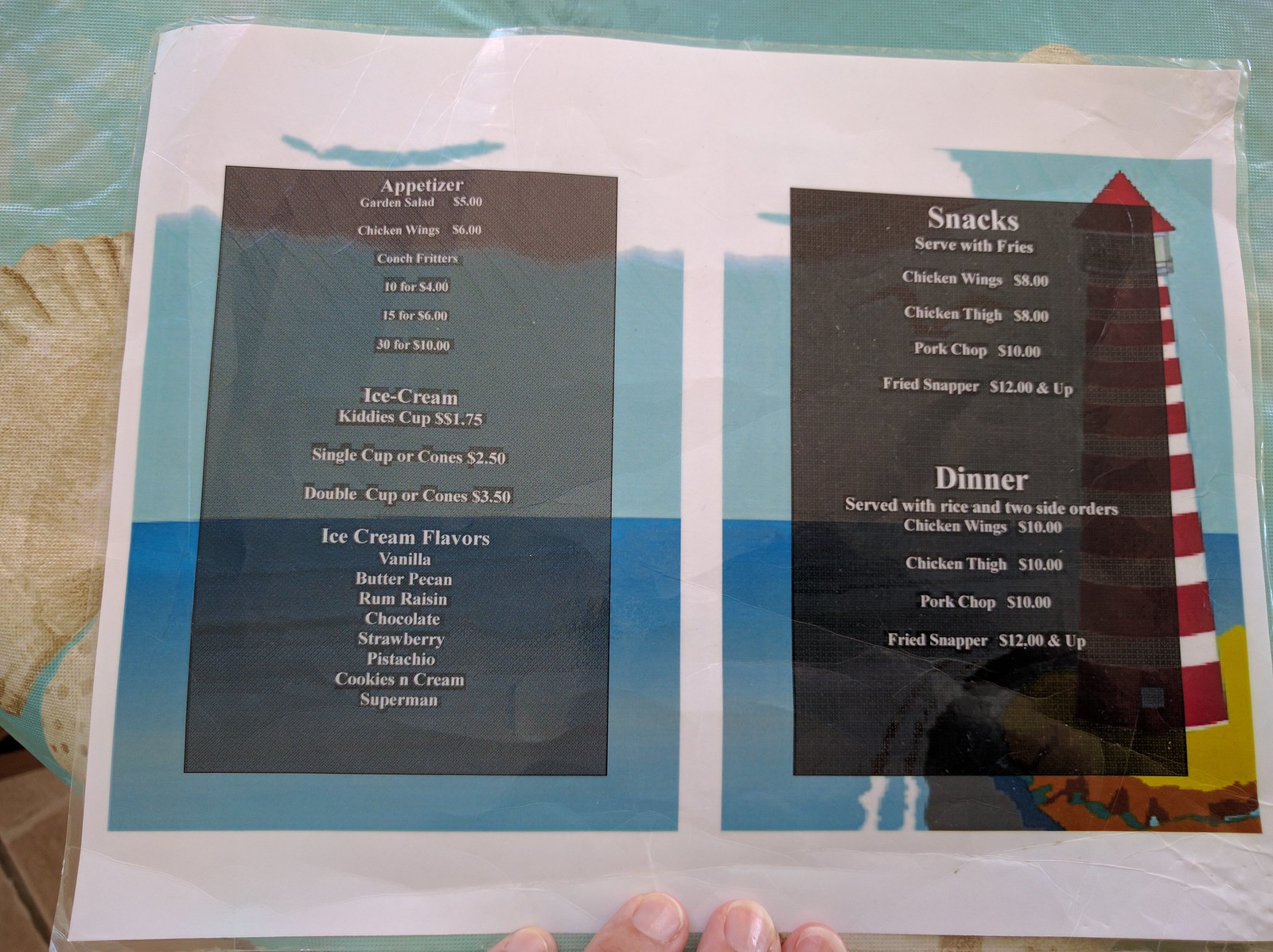The image features a laminated menu placed on what appears to be a tablecloth. On the left side of the image, there is a decorative element that resembles a brown shell, bordered by light blue and turquoise shades that evoke the impression of water. At the bottom of the image, the tips of four fingers of a white individual are visible, seemingly holding the menu in place.

The menu itself is distinctly outlined in white, with two blue rectangles displaying nautical imagery. The rectangle on the right side shows a red and white striped lighthouse against an ocean backdrop. Within these decorative borders, the main body of the menu is encased in a smaller black square with white lettering detailing the food items offered.

On the left side of the black square, the menu lists appetizers and ice cream options:
- **Appetizers:**
  - Garden Salad: $5
  - Chicken Wings: $6
  - Conch Fritters: $10 (for 4), $15 (for 6), $30 (for 10)

- **Ice Cream:**
  - Kitty's Cup: $1.75
  - Single Cup or Cone: $2.50
  - Double Cup or Cone: $3.50
  - Flavors: Vanilla, Butter Pecan, Rum Raisin, Chocolate, Strawberry, Pistachio, Cookies and Cream, Superman

On the right side of the black square, the menu details snacks and dinner options:
- **Snacks (served with fries):**
  - Chicken Wings: $8
  - Chicken Thigh: $8
  - Pork Chop: $10
  - Fried Snapper: $12 and up

- **Dinner (served with rice and two side orders):**
  - Chicken Wings: $10
  - Chicken Thigh: $10
  - Pork Chop: $10
  - Fried Snapper: $12 and up